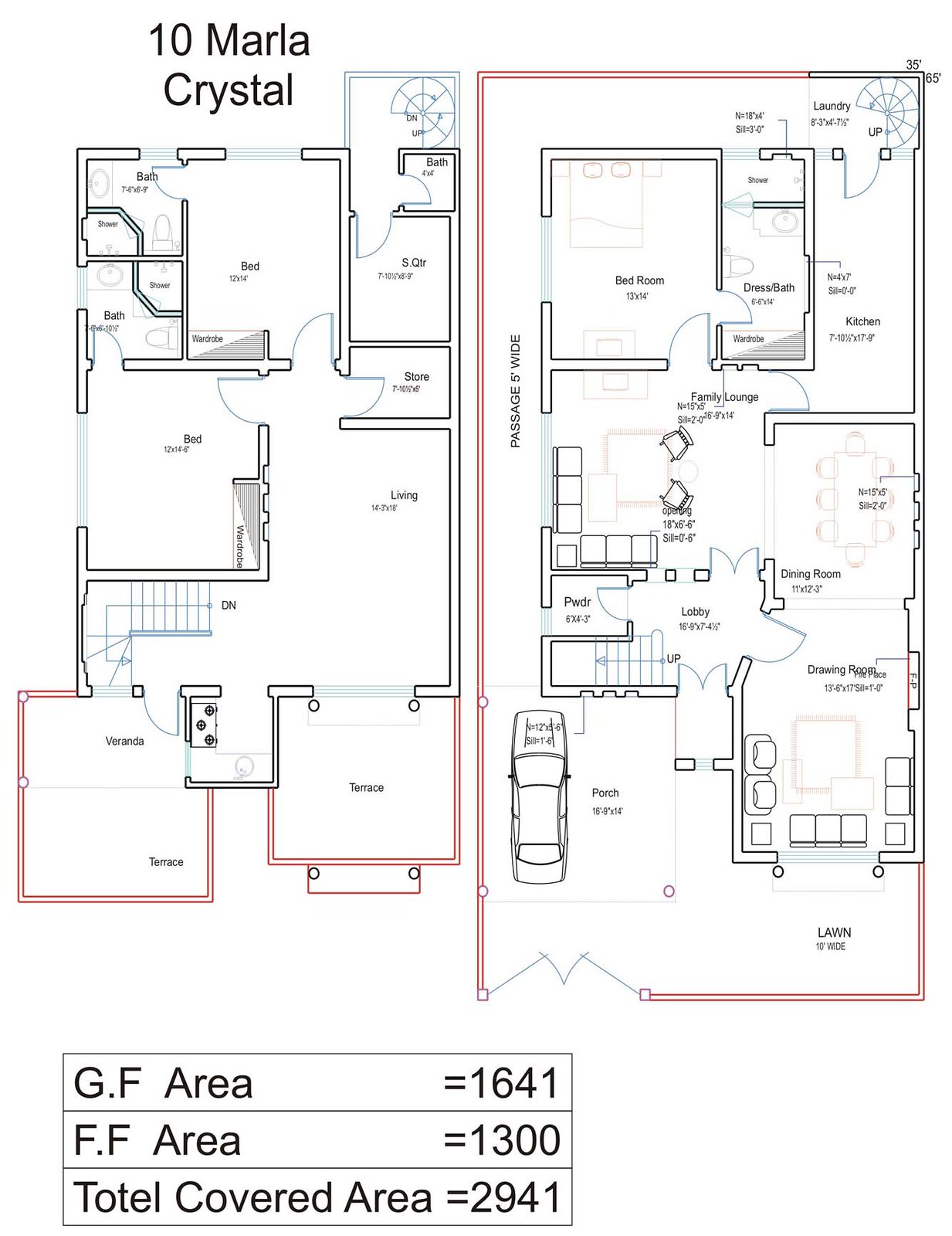This detailed blueprint depicts the architectural layout of a building labeled "10 Marla Crystal." The plan illustrates an expansive residential structure, potentially a large single-family house, segmented into various functional areas. The blueprint clearly delineates different rooms including multiple bedrooms, bathrooms, a living room, kitchen, and a porch. It also marks specific features such as the car parking area and a lawn, providing a comprehensive overview of the property's outdoor and indoor spaces. The lower section of the blueprint includes a chart detailing the area distribution: the ground floor (GF) spans 1,641 square feet, while the first floor (FF) covers 1,300 square feet, culminating in a total covered area of 2,941 square feet.